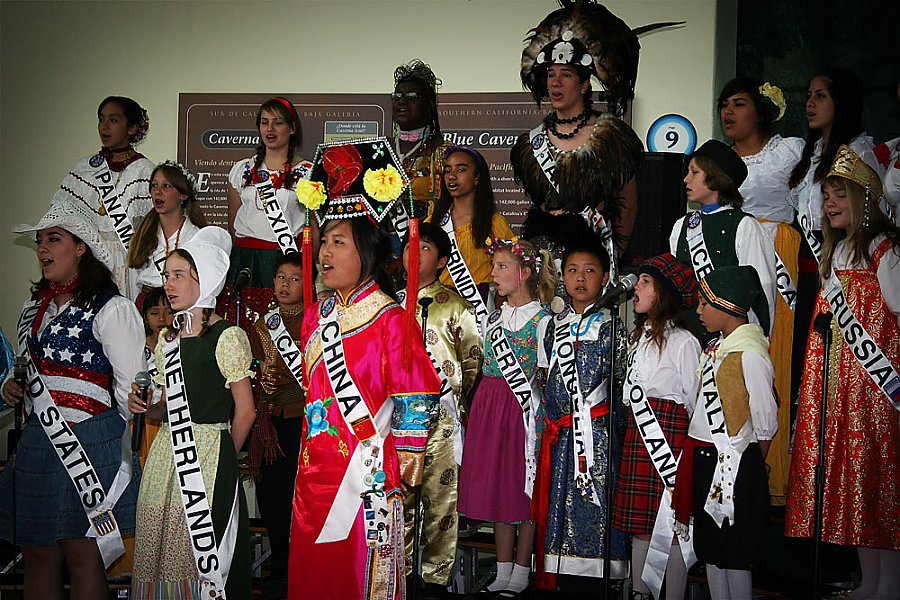This vibrant color photo captures a multinational group of approximately 20 children and teenagers, ranging in age from about 9 to 18 years old, adorned in their countries' traditional attire. They are lined up in three to four rows, facing forward with their mouths open, as if they are singing. Each child and teenager wears a white sash with the name of their respective country in bold black text. Notable countries represented include China, the Netherlands, the United States, Scotland, Italy, Russia, Panama, Mexico, and Germany.

A variety of colorful and distinct traditional outfits highlight the diversity on display. Among them, one can see a girl from the United States wearing a white cowboy hat, a vest decorated with the stars and stripes, and a white shirt. Next to her, a girl representing the Netherlands is dressed in a black outfit with white poofy sleeves and a round white hat. Another participant from China sports a shiny red silk dress paired with an elaborate black, yellow, and red headpiece akin to a kimono.

The setting appears to be indoors, and the presence of multiple microphones suggests they are performing, possibly singing, possibly celebrating global cultures through song. The image conveys a rich tapestry of international representation and cultural pride.